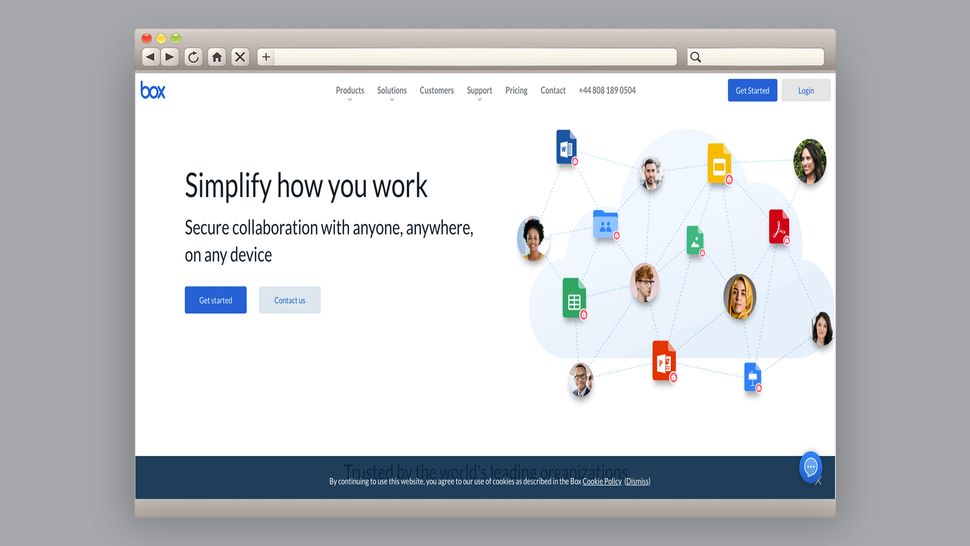The top left corner of the image displays a multi-colored bar with segments in red, yellow, green, and grey. Adjacent to this bar are icons including a left arrow, right arrow, refresh button, home button, and an X button. Below these icons, a large white rectangle is prominently featured, with a search bar inside it. The search bar contains the following text: "box, see products, solutions, customers, support, pricing, contact, 808-189-0504." 

Below the search bar, blue rectangles are labeled "Get Started" and "Login." Just below these buttons, there is a tagline that reads, "Simplify secure collaboration with anyone, anywhere, anybody." Additional calls to action, such as "Get Started" and "Contact Us," are also visible.

In the middle of the image, a visual network is depicted with a central blue square connected by lines to various icons, each representing different applications and tools: a network icon, a person icon, spreadsheet sheets, Acrobat, PowerPoint, and an unspecified icon.

At the bottom of the image, there is a disclaimer reading, "By continuing to use this website, you agree to our use of cookies as described," accompanied by a "Dismiss" button. Finally, on the far right side of the image, a blue circle contains a speech bubble with an ellipsis ("...").